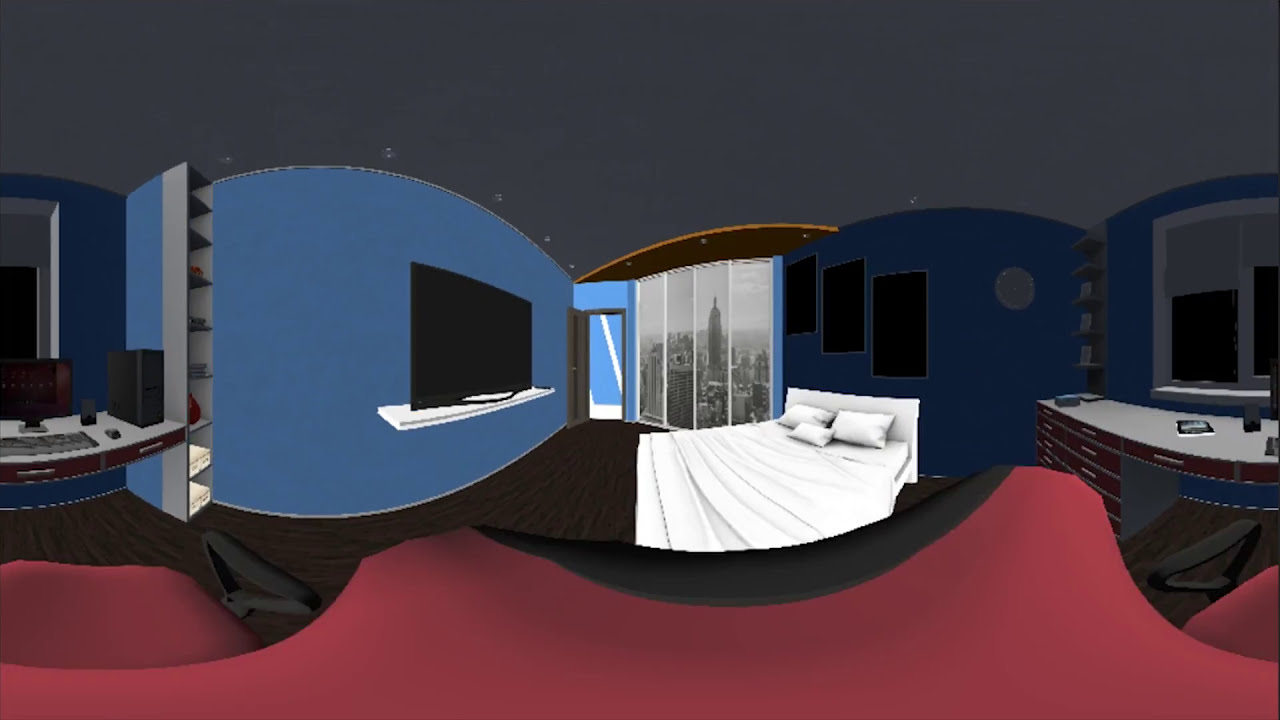The image is a highly detailed, computer-generated interior design model of a modern apartment. The bottom third of the image features an undulating maroon-colored floor border resembling carpet. Anchoring the center is a low-profile, white bed with a white headboard adorned with three white pillows. Directly behind the bed, a curved navy blue wall showcases a triptych of black panels. Flanking this feature, on the left, is a lighter blue curved wall holding a large TV monitor mounted on a white shelf. The right side of the image includes a sleek desk area, complete with a computer and additional shelving. A series of four window panels with a stunning city skyline view is centrally featured, adding depth and context to the space. The ceiling is a dark taupe brown, completing the sophisticated ambiance of the room.